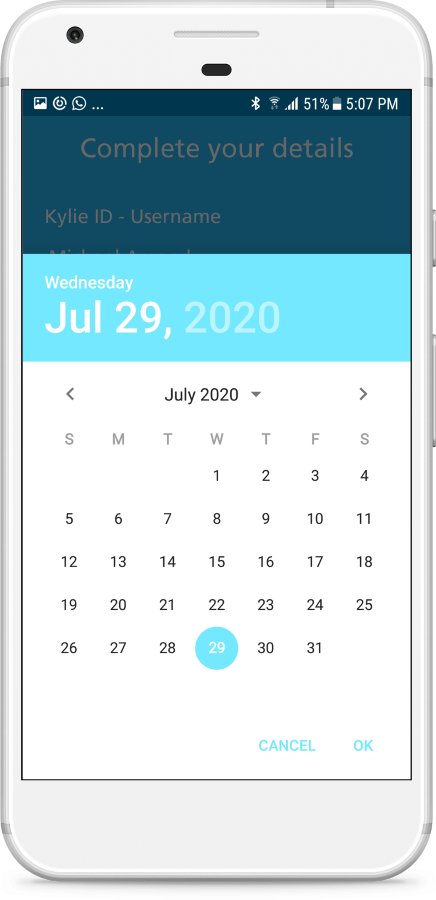This detailed caption presents a comprehensive description of the screenshot of a white phone's calendar app display:

"A detailed screenshot showcases a white phone's calendar app. At the top-right corner, the time is displayed as 5:07 PM alongside a battery icon indicating the phone is at 51% charge. The Wi-Fi and Bluetooth signals are active. The calendar, set to July 2020, specifically highlights Wednesday, July 29, with a light blue bubble encircling the date. A visible blue box at the top displays the date 'Wednesday, July 29, 2020,' complementing the selected date. At the bottom right, two blue buttons labeled 'Cancel' and 'Okay' are present, framed within the main interface.

Additionally, a grayed-out text at the top reads 'Complete your details,' followed by a white-font prompt for a 'Kylie ID username.' The phone's physical features are discernible—the black speaker positioned at the top center, a single black camera lens on the top-left, volume buttons, and an on/off button all located along the right side of the phone.

This precise depiction captures the minute and critical aspects of the screenshot, providing a clear, in-depth understanding of the image presented."